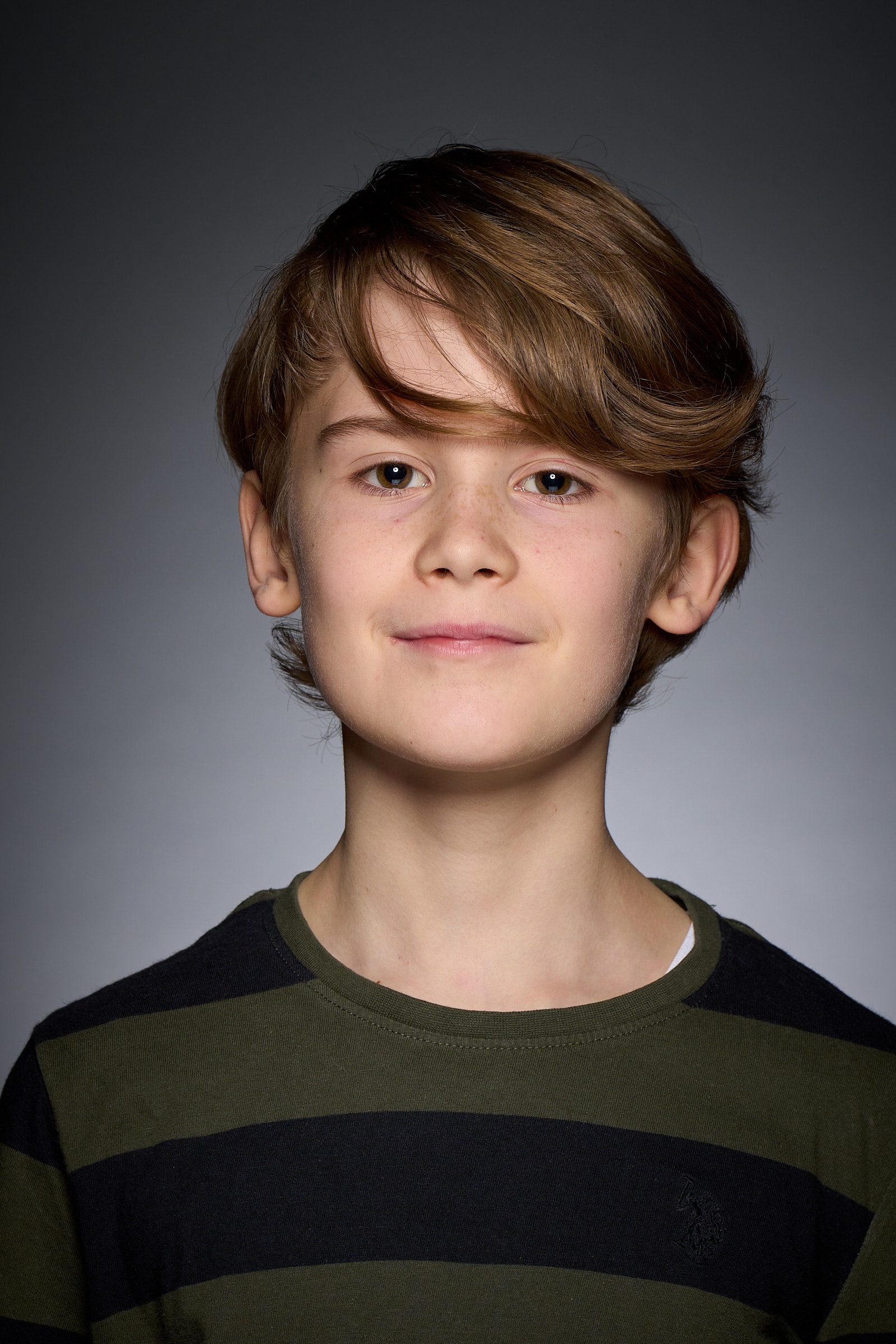This is a vertically oriented, full-color portrait of a young boy, approximately 11 years old, with a pale complexion. He has wavy, medium-length hair that is a combination of reddish-brown and light brown, styled with long bangs covering one eyebrow and shorter at the back. The boy is wearing a crew neck pullover top with olive and black horizontal stripes. His brown eyes are clearly visible, along with a few freckles across his nose. He has a semi-smile on his face, suggesting he is in good spirits and focused, likely posing for what appears to be a professionally taken school photo. The background features a gray gradient that becomes lighter towards the center, enhancing the subject's visibility. The young boy's relaxed and happy expression completes the charming, representational realism of the photograph.